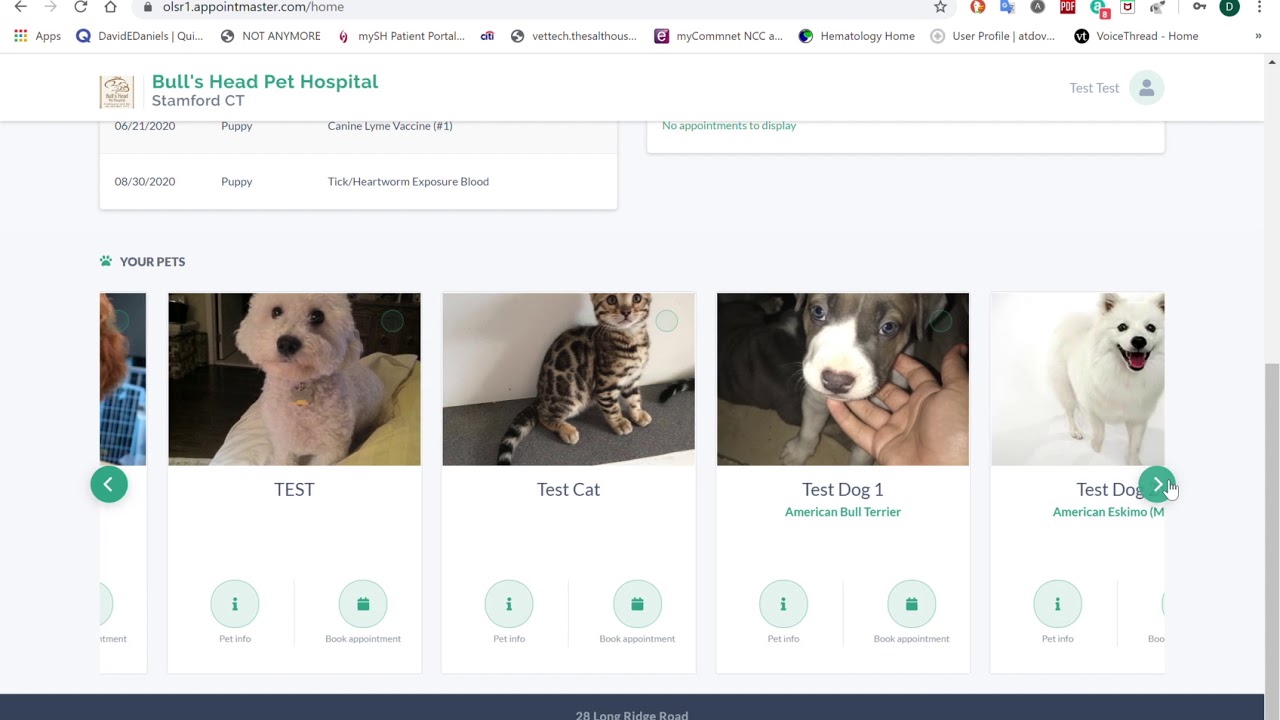The image features a partially cropped web browser, obscuring the top part of the screen. The visible URL is "olsr1appointmentmaster.com/home," flanked by several icons on the right. The bookmarks bar is populated with various links, including "David E. Daniels," "apps not anymore," "my sh patient portal," "vet tech," "the salt house," "my comment," "NCC hematology," "home user profile," and "voice thread home." Additionally, the bookmark "Bull's Head Pet Hospital in Stamford, Connecticut" is highlighted. Below, on what appears to be an appointment or test schedule, it lists:
- "06/21/2020: Puppy Canine Lyme Vaccine Number One"
- "08/30/2020: Puppy Heartworm Exposure Test"

The schedule also alludes to test results or appointments for "test cat" and "test dog one."